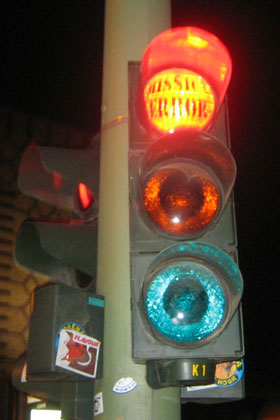This distinct nighttime photograph captures a traffic light attached to a steel pole, illuminated against a pitch-black sky. The traffic light has three lenses: the top one is red and illuminated, bearing an "ERROR" sign faintly visible in black text. The middle lens appears orange, and the bottom lens is an unexpected aqua blue. Each lens is framed in black with glare shades on top, resembling small hoods to diffuse the light. Underneath the lights, the pole features a black cylinder labeled "K1" in yellow text. To the left of this main traffic light, there’s another set of lights mounted on the same pole, oriented perpendicularly to the camera. The red lens of this secondary traffic light is also illuminated. Adjacent to the pole is a rectangular control box with a white sticker, the details of which are indiscernible, though it features a red design resembling a dragon. The photograph appears to be taken with a flash, causing slight reflections on the lenses of the lights.